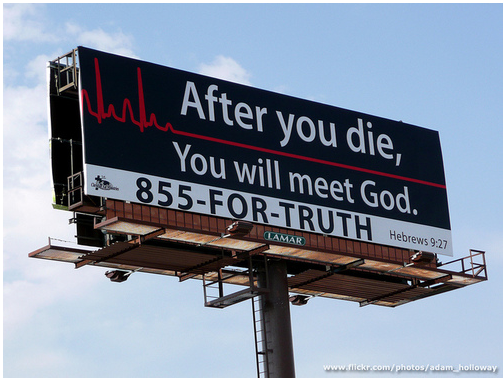The photograph captures a tall billboard set against a blue sky with scattered white clouds. The billboard is affixed to a long, cylindrical metal pole with an attached ladder. The main portion of the billboard features a stark black background with large white text stating, "After you die, you will meet God," punctuated by a red lifeline that has flatlined, symbolizing a heartbeat monitor. Below the main message, a white section displays the phone number "855-4-TRUTH" and a biblical reference, "Hebrews 9:27," in black letters. The bottom of the billboard shows the word "Lamar" in white letters set against a brown, rusted-look platform with a green background. The billboard is also equipped with lights on either side to illuminate the sign. In the bottom right-hand corner, a website, "www.flickr.com," is visible.